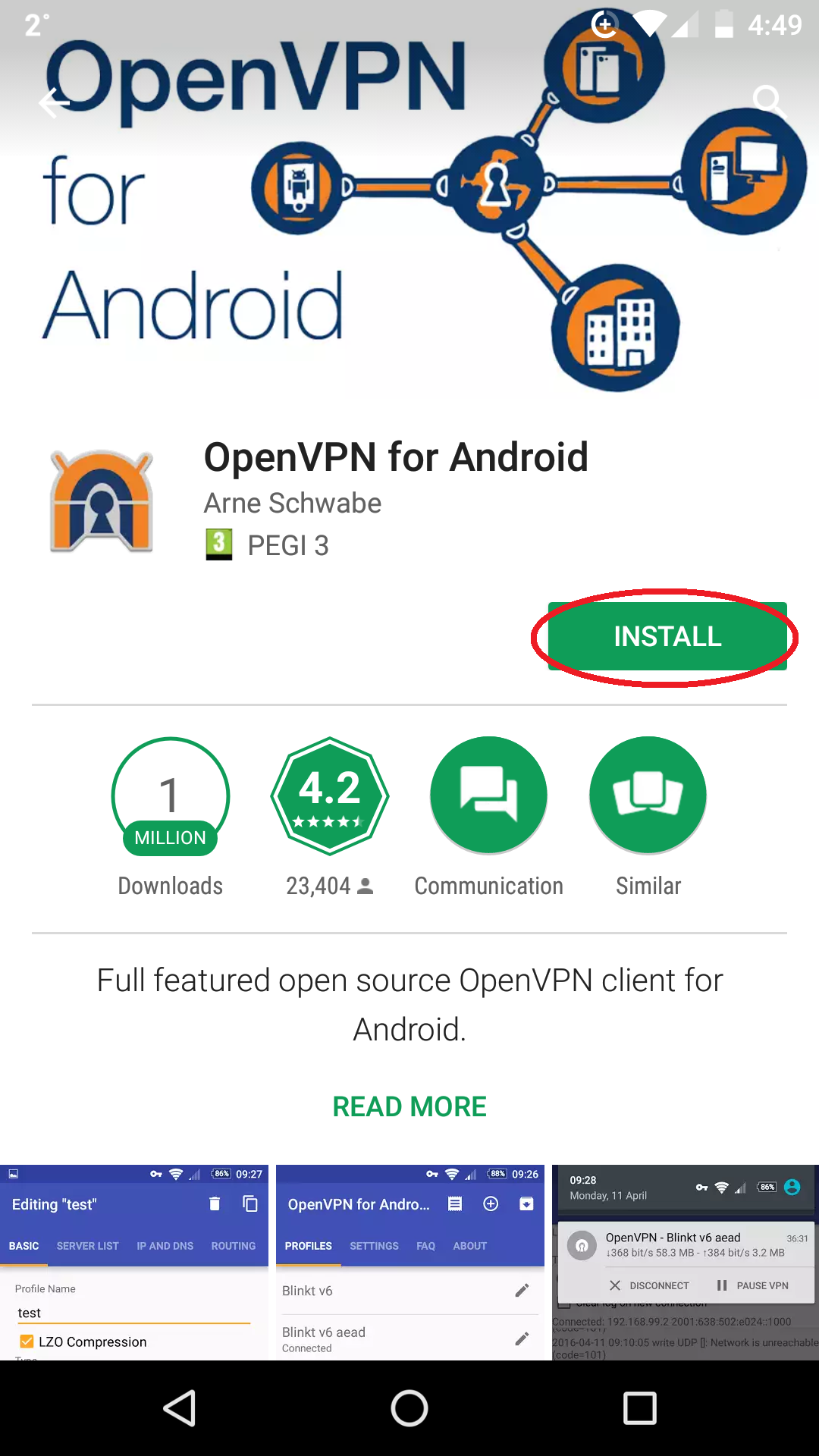The image depicts a screenshot of an Android phone displaying the Google Play Store page for the "OpenVPN for Android" app. The phone's status and navigation bars confirm it is an Android device. The app, developed by Arnie Schwab, is prominently featured with its title at the top followed by its PEGI 3 rating.

A green "Install" button is highlighted with a red, photoshopped circle emphasizing it. Just below this button, several statistics are displayed: the app has been downloaded over 1 million times, has an average rating of 4.2 stars out of 5, and has amassed 23,404 reviews. The reviews are categorized under "Communication" with a speech bubble icon, and next to it, another set of icons shows an extensive list related to the app’s features and functionalities. 

The detailed app description indicates that "OpenVPN for Android" is a full-featured, open-source VPN client for Android devices. A "Read more" button below the description provides additional information about the app. 

Further down, three screenshots of the app interface are displayed. Two of these screenshots feature a purple menu heading, while the third showcases a notification received upon downloading the app.

At the bottom of the screenshot, the Android navigation bar is visible with a home button, a back arrow, and a square button.